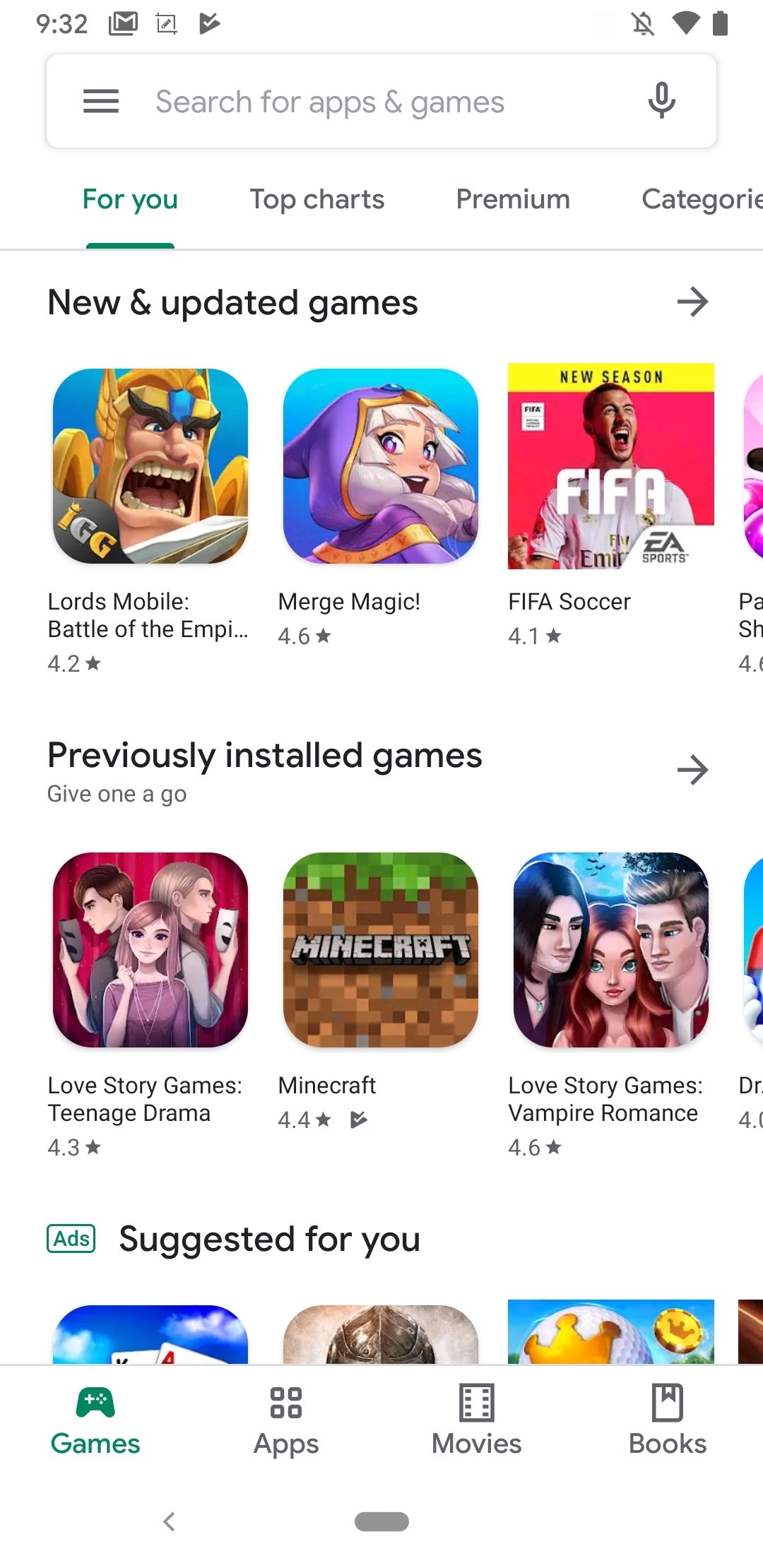A screenshot of a smartphone displays a white background with various interface elements. At the top right corner, the time is shown in gray as "9:32". Adjacent to it are several icons: a gray square with a white "M", a white square with a gray pencil inside and a gray border, a gray triangle with a white checkmark, a gray outlined bell with a strikethrough line, a gray Wi-Fi symbol, and a gray battery icon.

Below these icons is a white rectangle outlined in gray, containing three horizontal gray lines. Next to this is the text "Search for apps & games" in gray, followed by a gray microphone icon. 

Further down, there are four categories with a thin gray underline: the first is green and underlined, labeled "For you". The others are gray and labeled "Top charts", "Premium", and "Categories", though part of the "E" and the "S" in "Categories" are cut off.

A thin gray line stretches across the screen underneath these categories. Below this, in black text, it says "New & updated games" with a gray arrow pointing to the right beside it.

Listed games include:
1. "Lords Battle: Battle of the Empire..." with a rating of 4.2 stars.
2. "Merge Magic!" with a rating of 4.6 stars.
3. "Fight for Sakaar" with a rating of 4.1 stars.
4. A game partially cut off with "P-A-S-H".

Another section follows, titled "Previously installed games" with a gray arrow pointing to the right, followed by the prompt "Give one a go".

Listed previously installed games include:
1. "Love Story Games: Teenage Drama" with a rating of 4.3 stars.
2. "Minecraft" with a rating of 4.4 stars.
3. "Love Story Games: Vampire Romance" with a rating of 4.6 stars.
4. Another game partially cut off with "D-R" and a rating of 4.0 stars.